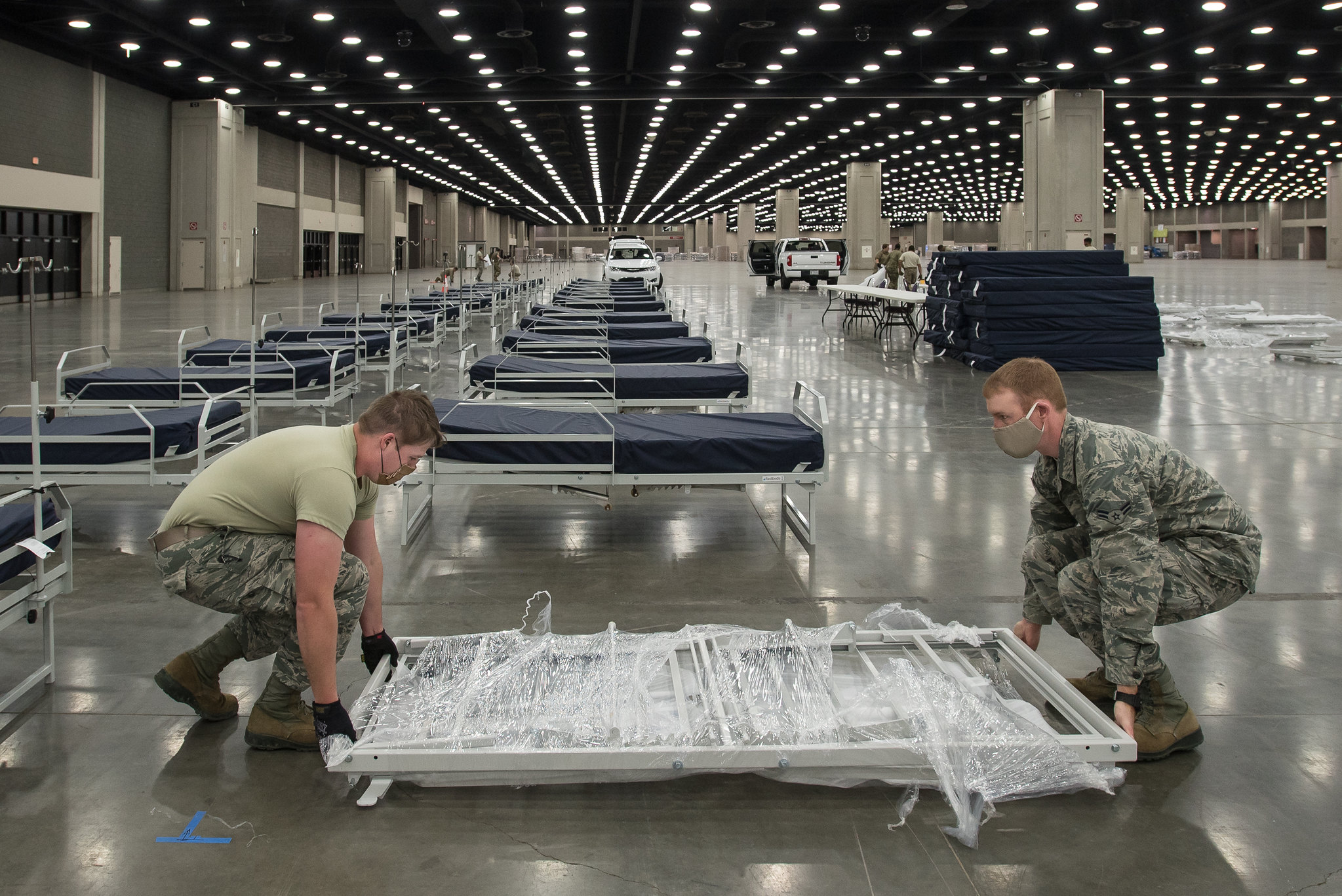The image depicts an indoor scene, likely set within a large conference center or parking deck area, where military personnel are setting up numerous cots. The setting has a cement floor and features multiple gray columns and a high, black ceiling with ventilation ducts and rows of round, white lights that reflect off the ground. The two soldiers, both wearing face masks, are in the process of assembling a metal cot that still has plastic shrink wrap around the frame. The soldier on the right is fully dressed in camouflage attire with brown boots, while the soldier on the left wears camouflage pants, a green t-shirt, and black gloves. In the background, dozens of cots with white frames and dark blue mattresses are neatly aligned in rows extending into the distance. Additional elements include vehicles such as a white pickup truck, another white vehicle, and people carrying items. There's also a long white folding table with black chairs, emphasizing the large-scale preparedness operation, possibly for an emergency shelter in response to a natural disaster.